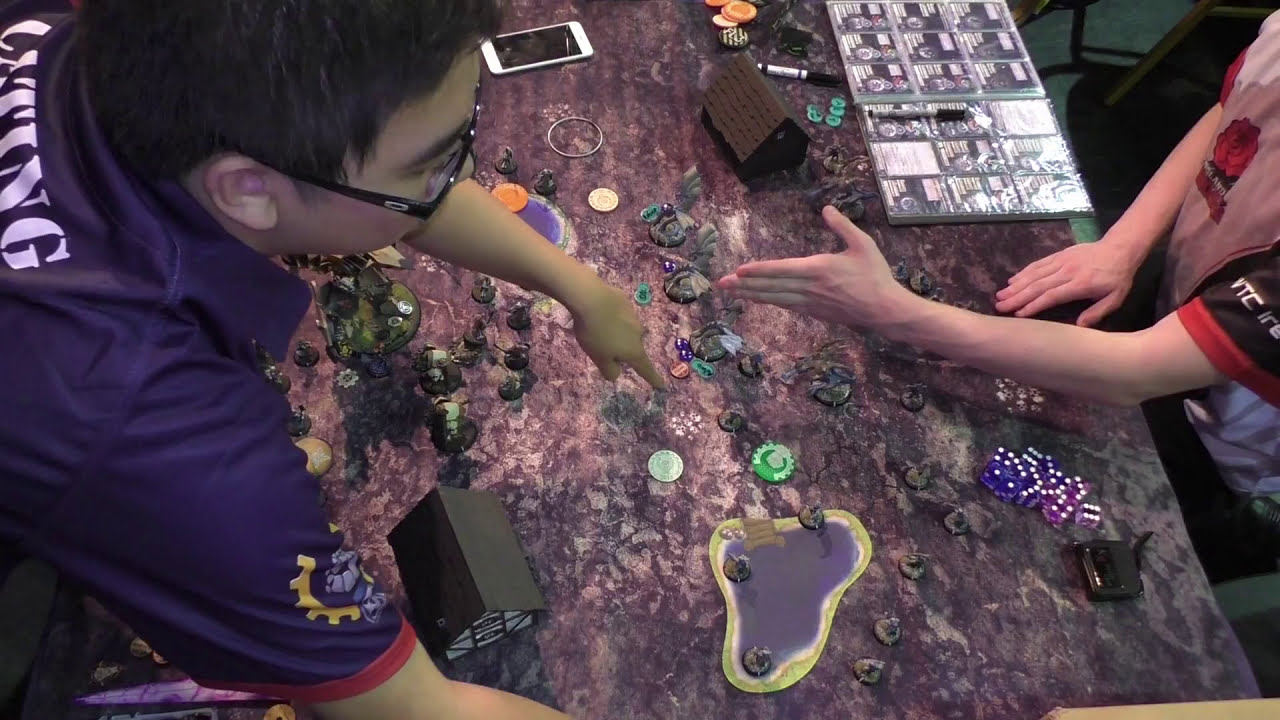The image features an overhead shot of a detailed table setup, likely for a tabletop game or a model display. At the center of the scene is a young Asian man with short black hair and black glasses, dressed in a navy blue t-shirt featuring a gold and blue logo on the sleeve and white text on the back. He appears to be intently examining the intricate model on the table, which includes small buildings, a lake, trees, and other architectural elements. Across the table, a partially visible individual, dressed similarly in esports attire, extends a hand toward the young man, possibly indicating a handshake or pointing gesture. The tabletop is cluttered with various game pieces, including an array of colored dice and what appears to be a marble-like surface. A white iPhone is also placed on the table to the far left. Additional hands and arms, likely belonging to other participants, are seen pointing towards the model, suggesting an interactive and possibly competitive environment.